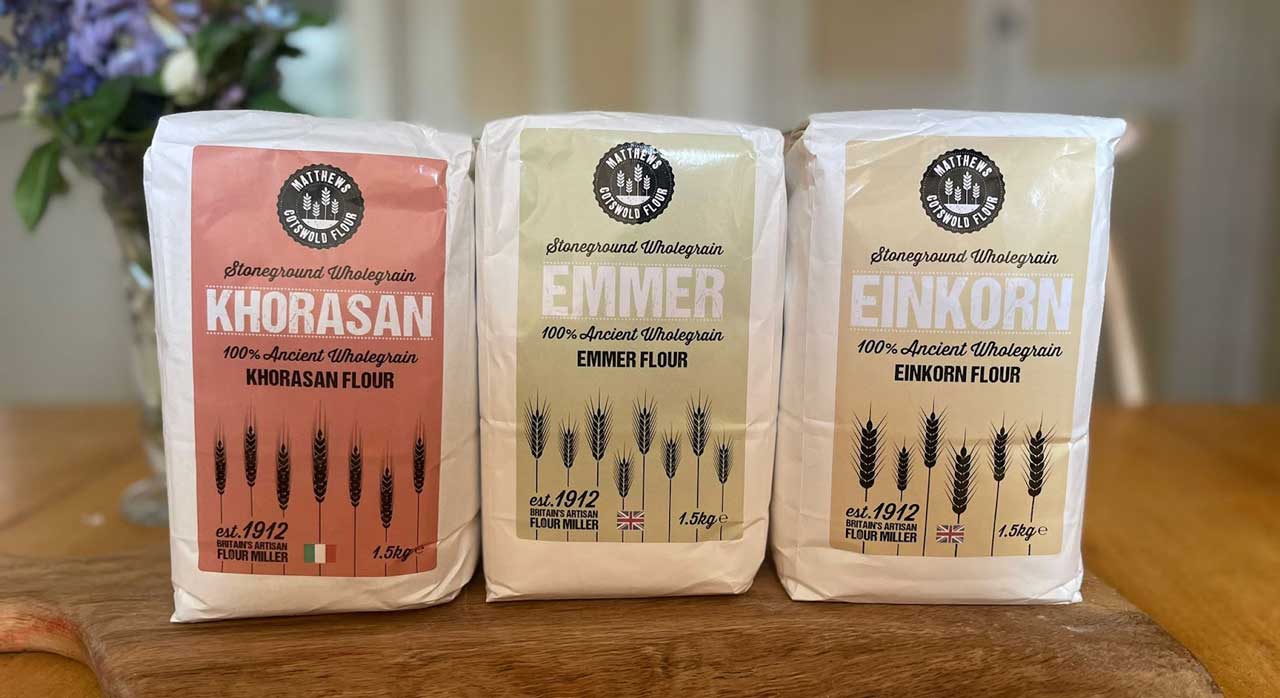In the image, three distinct packages of Matthews Flour, all weighing 1.5 kg, are displayed on a wooden trencher with a handle. The trencher rests on a wooden table. Each flour package is made of stone ground whole grain and is distinguished by its vibrant background color and type: the leftmost package, with a red background, is labeled Corazon Flour; the center package, with a light green or yellowish background, is Emmer Flour; and the rightmost package, with a light orange or peach-colored background, is Einkorn Flour. The top of each package proudly displays Matthews Flour's logo, along with the text "Established 1912" and "100% ancient whole grain flour." A detailed illustration of wheat adorns each package, reinforcing the stone ground whole grain message. In the background, though blurred, a vase with green leaves and purple flowers can be seen, partially obscured behind the leftmost flour bag, adding a touch of natural beauty to the setting.